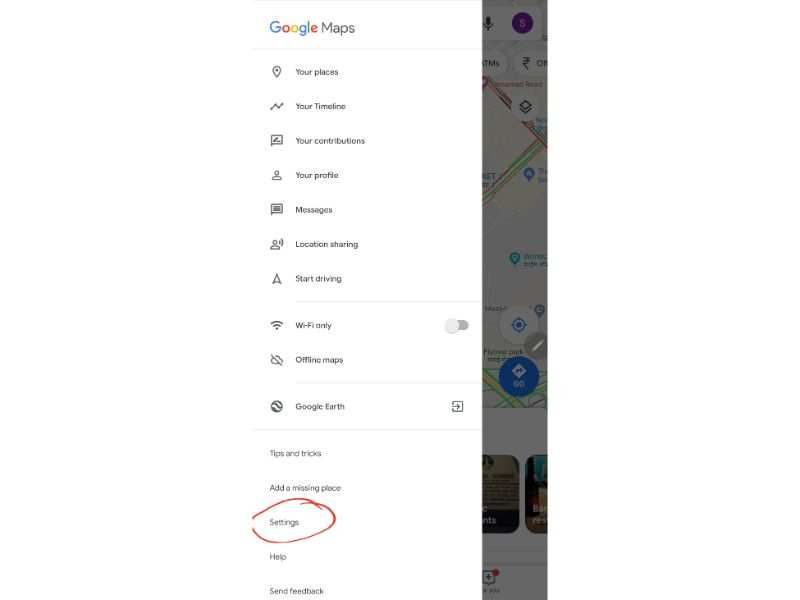The image is a detailed screenshot of the Google Maps app interface. 

On the left-hand side, a prominent vertical white sidebar occupies most of the space. At the top left corner, the familiar "Google Maps" branding is displayed, showcasing the iconic Google colors on the word "Google." Below this, a vertical menu bar presents various options: "Your places," "Your timeline," "Your contributions," "Your profile," "Messages," "Location sharing," and "Start driving."

Following this sequence, a thin gray dividing line appears. Beneath it, the menu continues with "Wi-Fi only," which shows a slider toggled off, hence displayed in gray. The list then proceeds with "Maps" and includes additional gray dividers before listing "Google Earth," "Tips and tricks," "Add a missing place," "Settings," "Help," and "Send feedback." Around the "Settings" option, a crudely drawn red circle encircles it, likely made using a basic drawing tool.

On the right side of the image, part of a Google Maps map is visible, muted by a gray filter overlay. The map section displays several intersecting streets and avenues. Additionally, a blue "Go" button is prominently featured, accompanied by a series of smaller images lining the bottom of the screen.